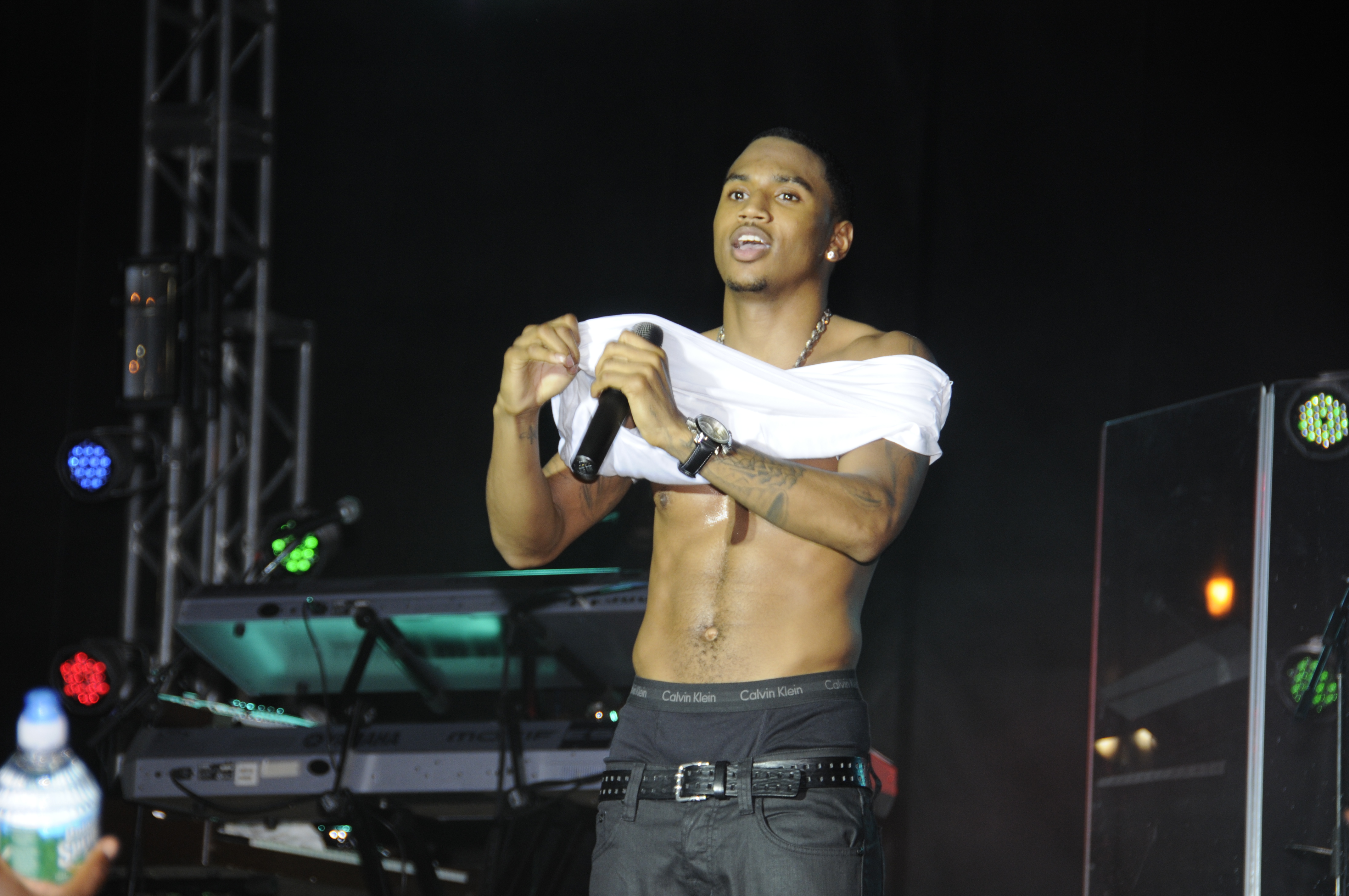The dynamic image captures the renowned singer Trey Songz in the midst of an electrifying performance on stage. Positioned at the center, Trey is energetically peeling off his white t-shirt, revealing his sculpted chest and black Calvin Klein underwear as his black pants hang low. His open mouth suggests he’s either mid-song or engaging with the audience, his gaze fixed on the crowd. Trey, an African-American man with short hair and a thin black beard, accessorizes with a gleaming chain around his neck and an earring. He grips a microphone in one hand while a watch adorns one arm, indicating his readiness for an intense performance. The stage is bustling with essential concert apparatus including lights, sound equipment, a DJ table, keyboards, and speakers. The colorful spectrum of black, white, brown, blue, green, red, yellow, and orange illuminates the scene, enhancing the vibrant ambiance. In the bottom left of the photo, a hand holding a water bottle subtly enters the frame, adding a touch of behind-the-scenes realism to what is likely a shot from a professional live concert.